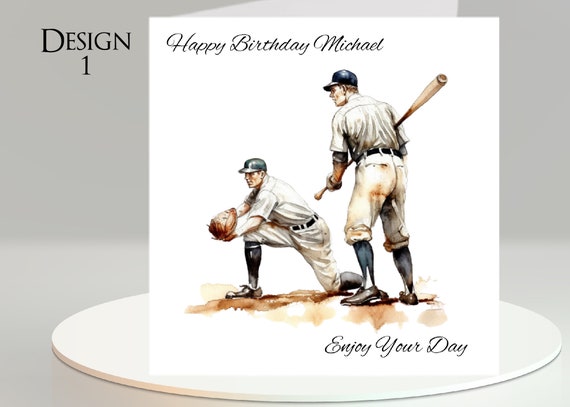The image is of a thoughtfully-designed birthday card set against a gray background. The card prominently features two male adult baseball players dressed in classic white uniforms with tall blue socks, dark blue baseball caps, and leather shoes. One player, positioned as the catcher, is bent down with a glove in hand, while the other player, the batter, stands poised with a long bat. The scene evokes a nostalgic, old-school baseball vibe. 

At the top left corner of the card, written in elegant script handwriting, it says "Happy Birthday, Michael," and the bottom right corner bears the message "Enjoy your day," also in black cursive font. The card appears to be propped open slightly, revealing its white interior. The entire card rests on a circular white platter, contributing to the card's clean and classic aesthetic. The design elements and minimalistic color scheme of white, gray, and dark blue lend it a refined and timeless look.